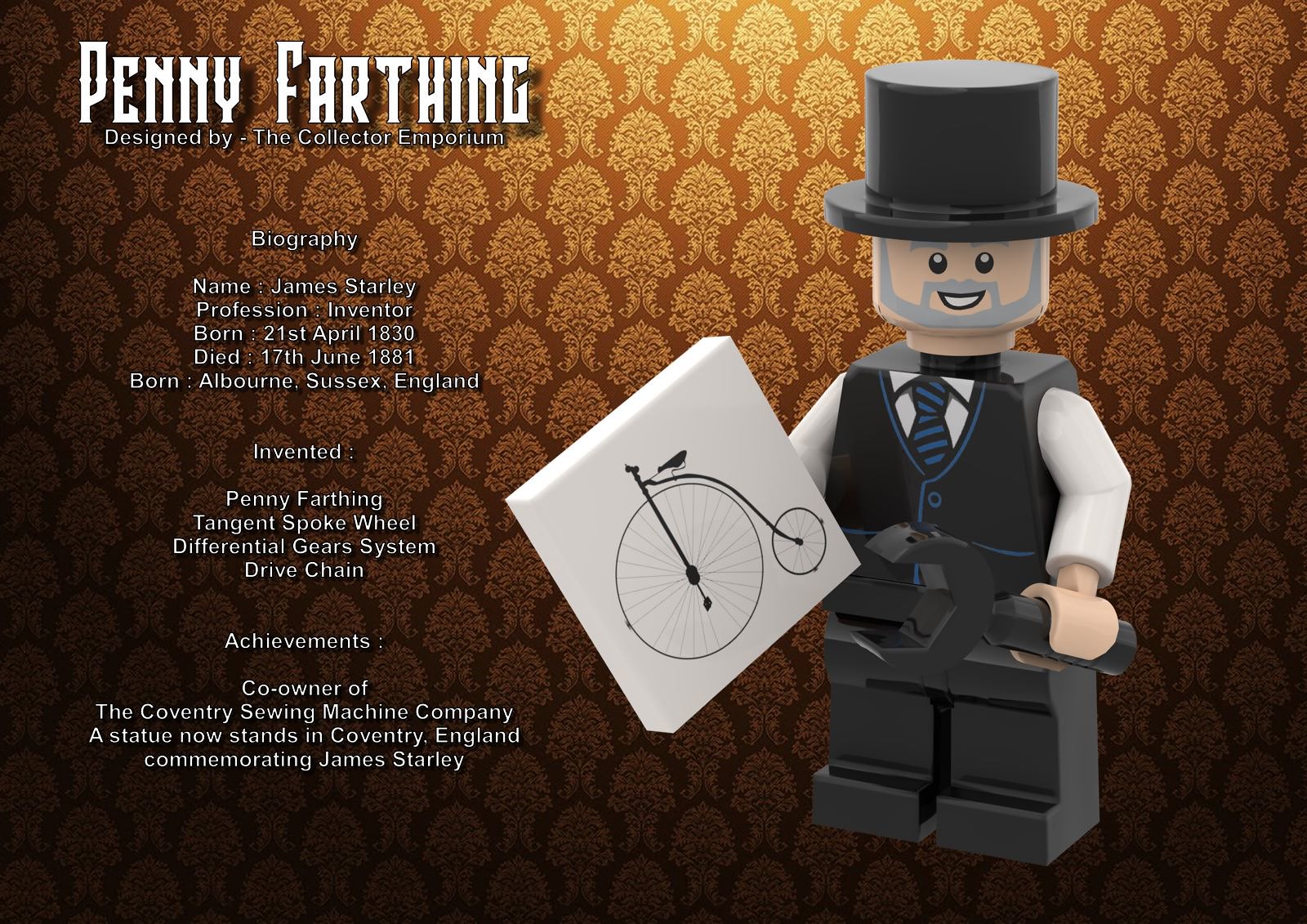The image features a highly detailed digital presentation with a richly textured brown and gold background adorned with flowery etched symbols. On the left side, the text in white letters reads "Penny Farthing, designed by The Collector Emporium," followed by a detailed biography of James Starley, an inventor born on April 21, 1830, in Albourne, Sussex, England, and who died on June 17, 1881. His achievements include inventing the Penny Farthing, the tangent spoke wheel, the differential gear system, and the drive chain. He also co-owned the Coventry Sewing Machine Company, and his legacy is honored with a statue in Coventry, England.

On the right side of the image stands a miniature Lego character, whimsically detailed with a gray beard, mustache, and sideburns, dressed in an old-fashioned white shirt, black vest with blue piping, black pants, and a blue tie. The Lego figure sports a top hat and holds a Lego wrench in its left hand, while its right hand holds a drawing of an old-fashioned Penny Farthing bicycle, recognizable by its large front wheel and small rear wheel. The Lego figure smiles cheerfully, adding a playful touch to this informative and visually engaging presentation.